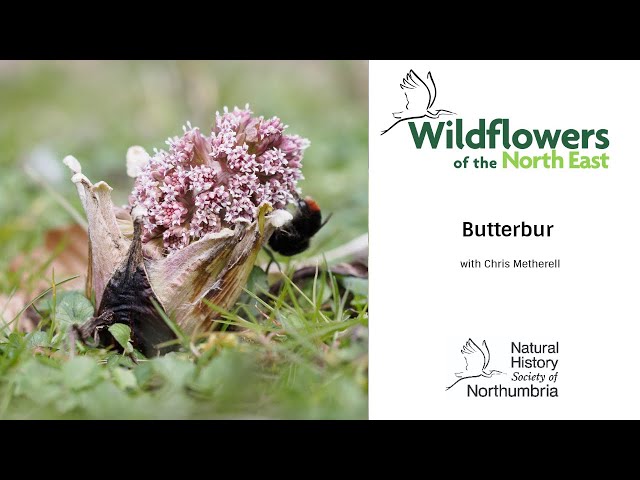This is an image, possibly a still frame from a video or the cover page of a report or presentation, titled "Wildflowers of the Northeast." The image features black bars at the top and bottom to fit the screen ratio. The left side displays a close-up photo of vibrant, pink wildflowers resembling a cluster of tiny blooms shaped like a pine cone or egg, growing from the damp, grassy forest floor amidst some weeds. A black and red-headed hummingbird is captured mid-flight, its beak diligently seeking nectar from one of the flowers. The background is artistically blurred to emphasize the subject. The right side of the image is dedicated to text on a white background, showcasing green text that reads "Wildflowers of the Northeast" with a black illustration of a crane flying over the 'W.' Below, in black text, it states "Butterbur with Chris Metherill," and is credited to the "Natural History Society of Northumbria," accompanied by a repeated black crane logo.